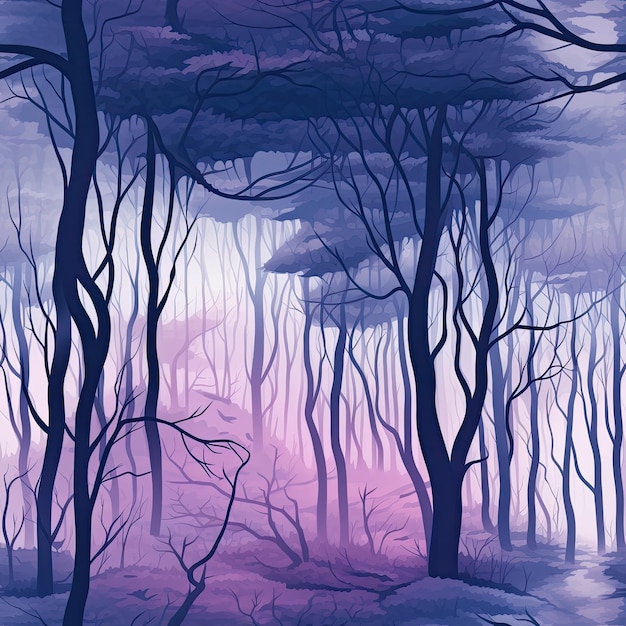This digital painting, with a somewhat cartoonish and animated style, depicts an exaggerated, atmospheric forest scene. The tall, spindly tree trunks, rendered in dark blacks and purples, stretch upward to a canopy of dark blue and purple foliage, giving the scene a ghostly, almost haunted appearance. The background transitions from a light grayish-purple to light blues and deeper purples, creating a flowing, misty ambiance that suggests the viewer is moving toward sunlight. The bare branches of the trees emphasize the ethereal, otherworldly quality of the forest. The ground mirrors these colors, with shades of light and dark purple, enhancing the overall moody and spectral feel of the image. The muted blues and purples, combined with the dark, bold lines of the tree trunks, contribute to a cohesive and intriguing woodland setting.